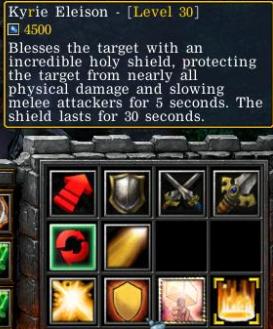This image is a screenshot from a medieval-themed crafting video game featuring a detailed endgame inventory and item description. The top half of the image is dominated by white text that reads "Kyrie Eleison, level 30," followed by a detailed description: "Blesses the target with an incredible holy shield protecting the target from nearly all physical damage and slowing melee attackers for 5 seconds. The shield lasts for 30 seconds." Next to the text, there is a symbol and the number "4,500" in gold font. The bottom half displays three rows, each containing four square slots with various items, including a red arrow, silver shield, two swords, a dagger, two circling arrows, a beam of light, an explosion, a yellow shield, a hammer, and a ring of fire. The layout is framed by a stone castle fortress design, with two of the squares highlighted in black. The interface blends a medieval fantasy aesthetic with a functional inventory system, typical of many strategy and role-playing games.